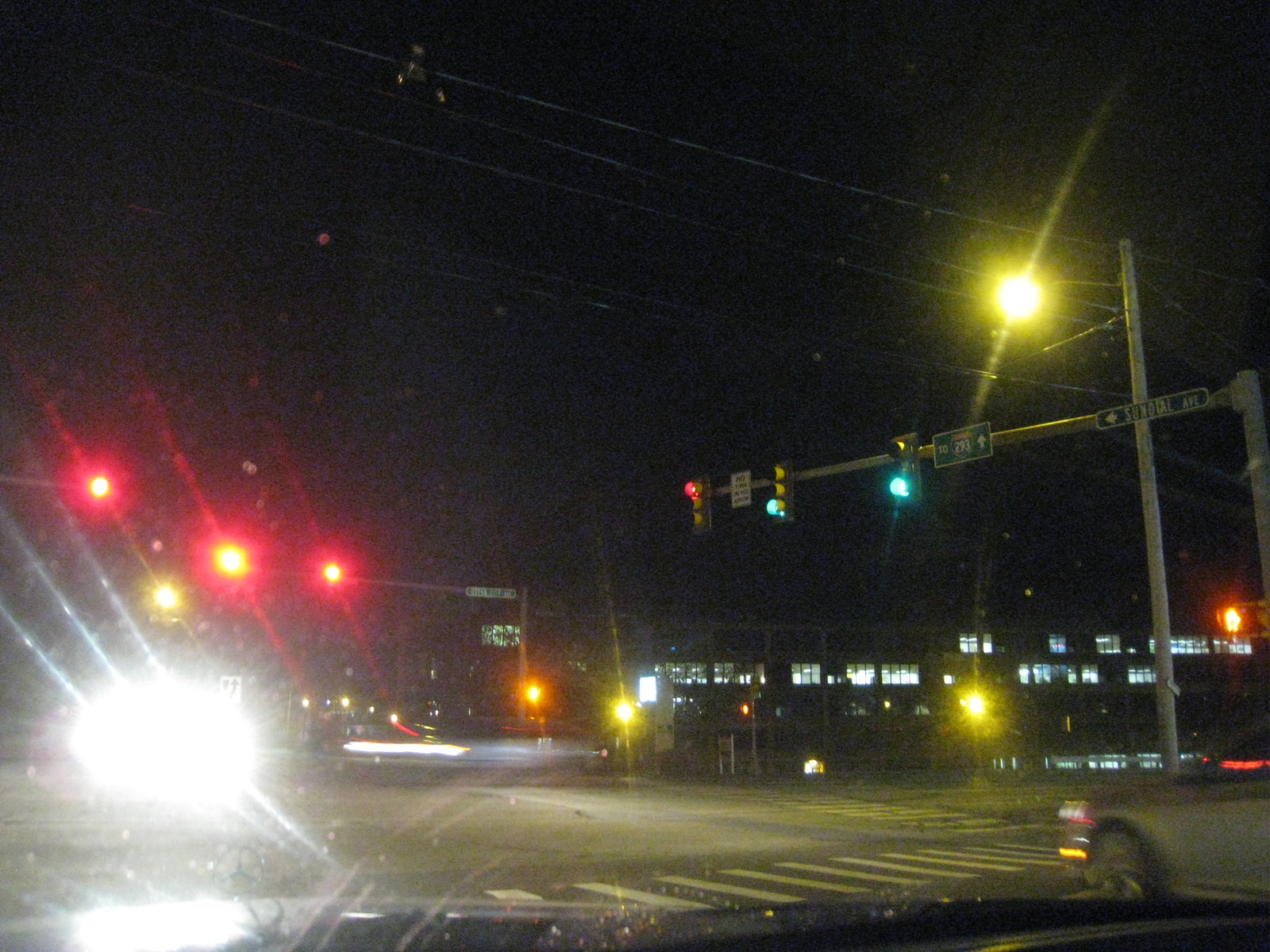A nighttime photograph captures a city intersection from the perspective of someone sitting at a stoplight. In the foreground, three red traffic lights hang prominently, indicating that the viewer's vehicle is angled at the junction. A gray car is visible on the right side of the frame, waiting at the light. The background reveals an office building with various lights illuminated in the windows, adding a sense of urban activity. A street sign reads "Sundial Avenue" as it intersects the main road, above which a sign for "295" is posted. Mounted on the same pole, two traffic lights shine green, while the one on the left displays red. The interplay of lights and urban structures creates a moody, nocturnal scene.